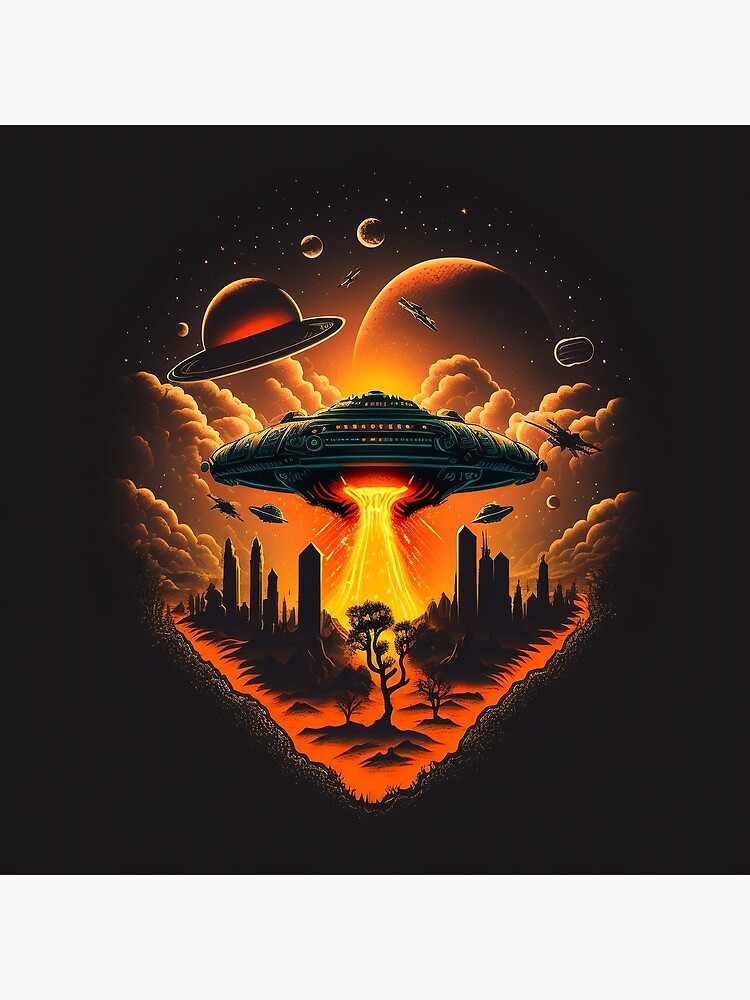The image is a square, computer-generated graphic set against a solid black background portraying a dramatic science fiction scene. Central to the composition is a large, dark spaceship adorned with gray and brown sections, peppered with small, square-shaped orange lights. This imposing mothership hovers over a city, emitting a brilliant beam of light downward onto orange-tinted ground. The illuminated scene reveals diagonal rows of buildings, forming a V-shape, flanked by sporadic trees. Above the spaceship to the upper left, a planet reminiscent of Saturn with its distinct ring glows in shaded hues of black and orange. The sky is dotted with smaller celestial bodies and a scattering of white specks representing stars. Complementing the primary spaceship are smaller ships, seemingly part of the invasion. The entire scene, highlighted with minimalistic colors like black, orange, white, and yellow, vividly illustrates the mothership's formidable presence and the futuristic cityscape beneath, showcasing a classic UFO, sci-fi aesthetic.